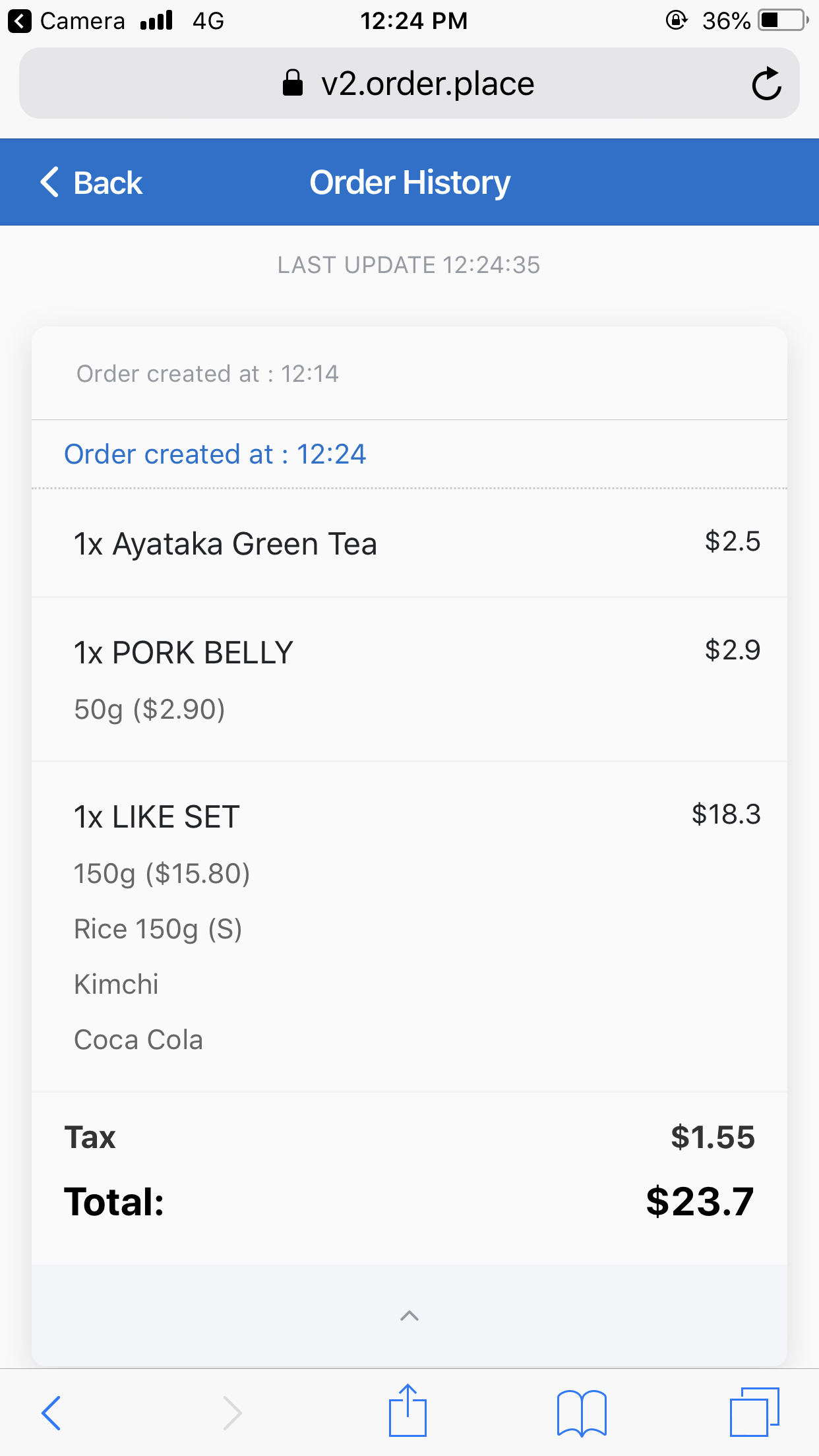The image depicts a screenshot of a mobile application interface resembling a cell phone display. At the top of the screen, the status bar reads "Camera" followed by "4G" and displays the current time "12:24 PM" with a battery icon at "36%", all in grey. Directly below the status bar is another grey rectangle containing a lock icon, the text "v2.order.place," and a refresh arrow.

Below this, a blue rectangle features a left-pointing arrow and the word "Back," next to which is the label "Order History." Underneath in grey text, it reads "Last update 12:24:35." The interface continues with two rectangular segments: the first is outlined in grey and states "Order created at 12:14," while the second is outlined in blue, indicating "Order created at 12:24."

Below these segments is a column listing various items including "1X AYATAKA green tea" and "1X PORK BELLY." Adjacent to each item on the right are their corresponding prices: "2.5," "2.9," "18.3," and "1.55" respectively. The list concludes with additional items such as "rice," "kimchi," and "coca cola," followed by tax details and a total amount of "23.7."